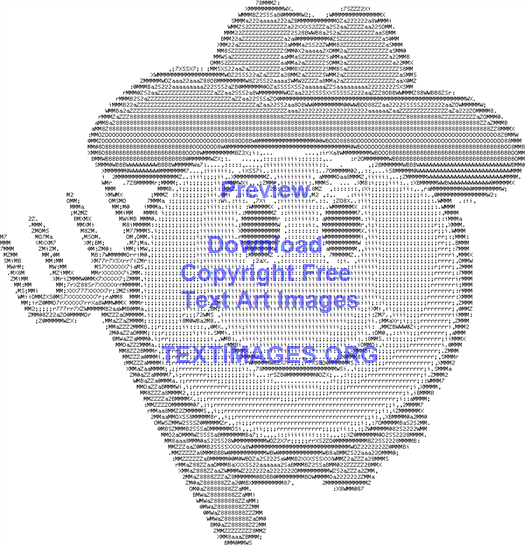The image is a pixelated, computer-generated smiley face that resembles a classic emoji. The smiley face features expressive, downward-turned eyebrows, large black oval eyes, and a broad smile. It is wearing a cowboy hat with a distinct "O" in the center. The face also has a little handkerchief or bandana around its neck. To the left of the smiley face, there is a gray pitchfork with four tines. The background of the image is white, and there is a light purple watermark that reads "Preview, Download, Copyright Free Text Art Images" along with the URL "textimages.org" printed in capital letters across the face, though it's not centered. The overall image appears grainy, emphasizing its pixelated nature and grayscale design.